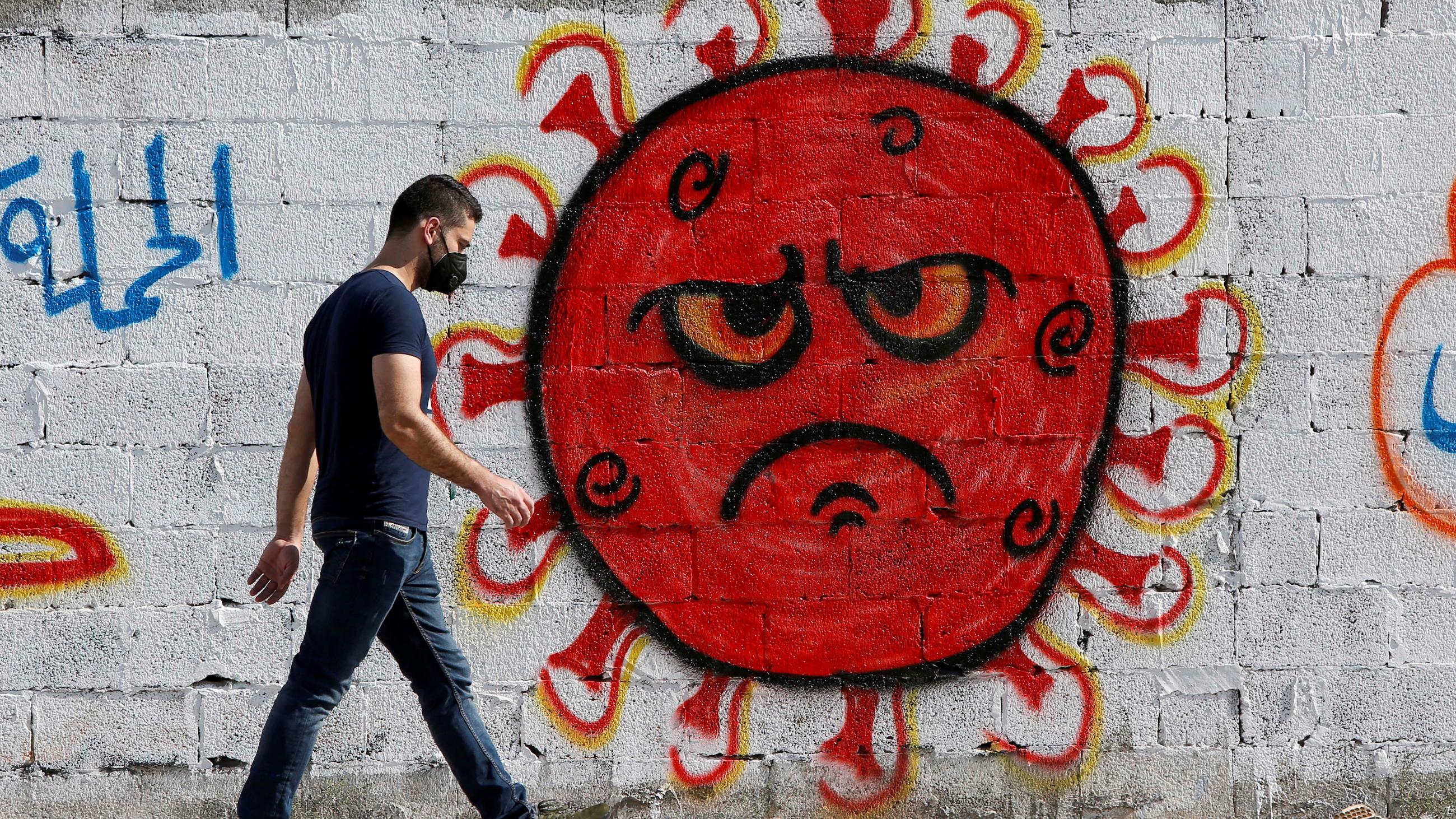This is a horizontally aligned rectangular image of a man, clearly visible from the side, walking in front of a white stone wall made of large cinder blocks. The man, who has short brown hair and wears a black medical mask looped around his ears, is dressed in blue jeans and a tight-fitting, short-sleeve dark blue t-shirt. He is on the left side of the image, looking down as he swings his arms while walking. Prominently featured on the white stone wall to his left is a large, painted sun with a distinctly expressive face. The sun, outlined in black and shaded with orange and yellow hues, sports a serious or angry expression with frowning mouth and glaring black-outlined eyes. The sun is surrounded by red and yellow curved rays. Additionally, some blue writing is visible on the upper left side of the wall, although its exact meaning is unclear. The overall atmosphere of the scene is bright and sunny.